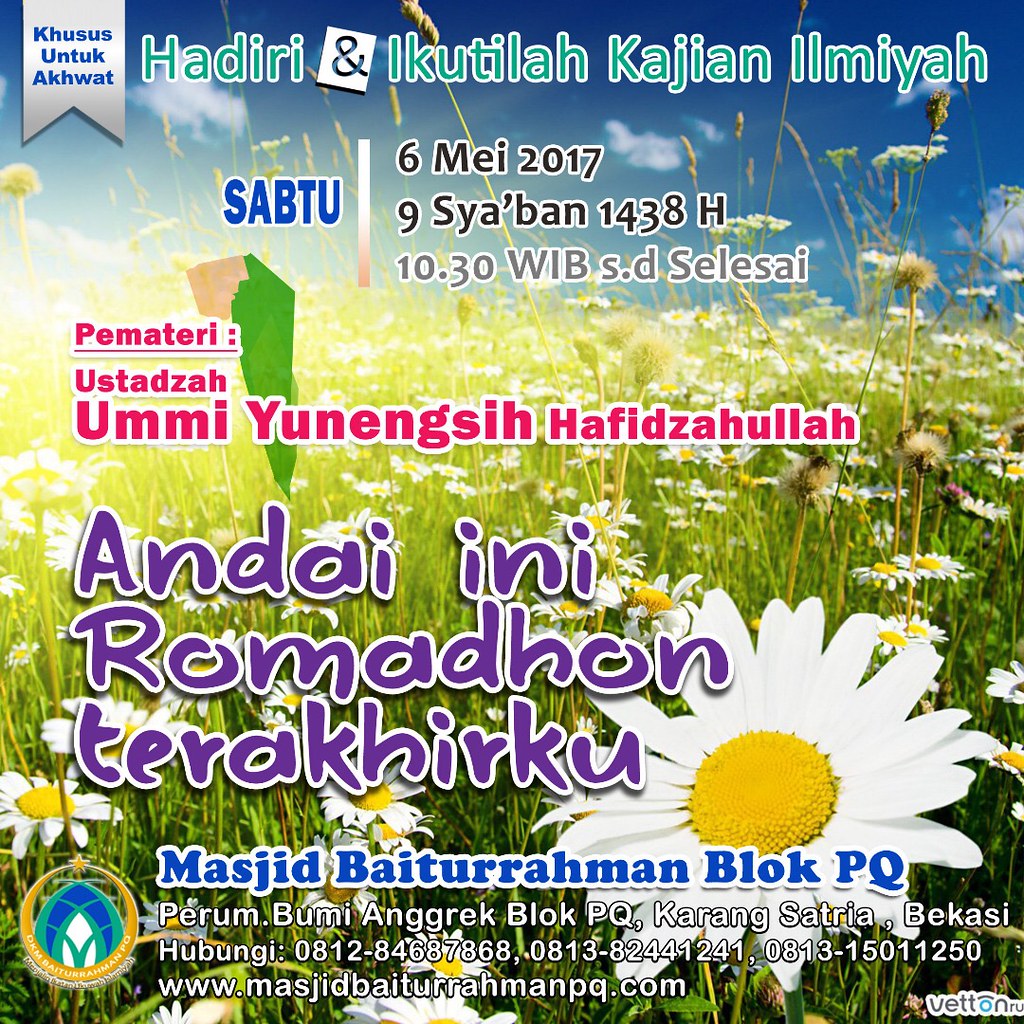The image is a flyer set against an outdoor scenic background depicting a vast field of daisies, characterized by their white petals with yellow centers, and vibrant green stems. Above this charming floral landscape, a serene blue sky filled with fluffy white clouds stretches across the top of the image. Dominating the top section of the flyer, there is a heading in green text with a white outline, saying "Hadiri and Iqtala, Qajian, Yemiya." Below this heading, in pinkish-red font, additional information is provided, and further down, a large, bold purple font adds prominence to more text. Moving towards the bottom, blue text outlines specific details, including "Masjid Baturaman Block PQ" and company-related information. Below this, in white text, contact details and the organization's website, www.masjidbaturamanpq.com, are clearly listed. Accompanying the text, at the bottom left, is a gold circular logo featuring a star at the top and a blue and green emblem inside, resembling a plant. The overall language appears to be a foreign, Eastern Bloc or Uzbekistani language, contributing an exotic aspect to this event flyer.